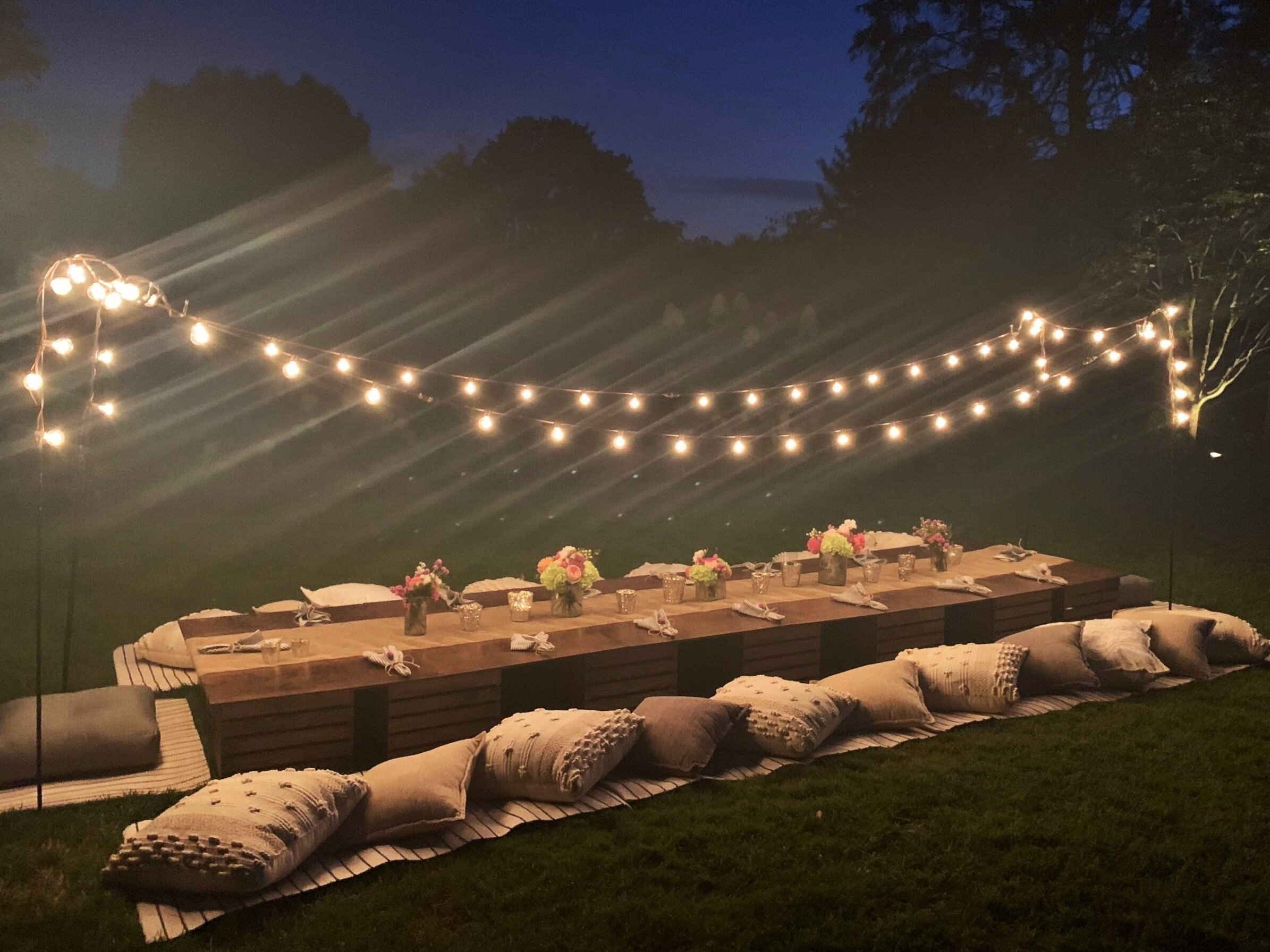This photo captures an outdoor evening garden setting with a charming and rustic table arrangement. An elongated table, positioned atop a low stone wall adorned with horizontal burlap sacks, is set for fourteen place settings (seven on each side). A beige table runner lies along the center of the table, topped with four elegant flower centerpieces. The seating consists of pillows set on top of carton boxes, adding a cozy vibe. Illuminating the scene are two rows of string lights suspended on poles, casting a warm glow over the entire setup. The backdrop reveals a stone pit on the left side of the table and a mountainous, tree-lined horizon with tall peaks, against a dark blue night sky.